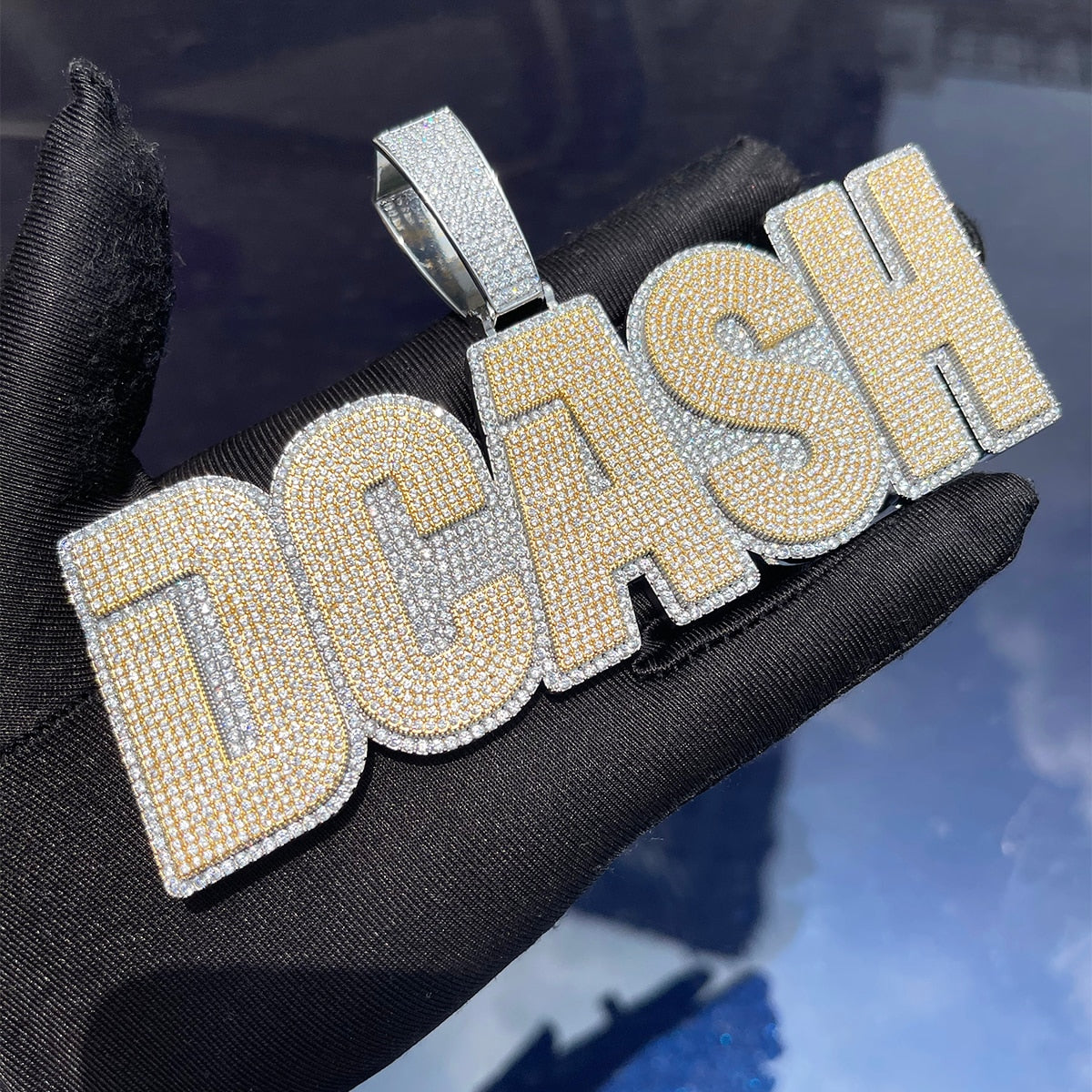The image is a close-up, in-color photograph depicting a hand wearing a black latex glove, holding a large, glittering pendant. The pendant spells out "D CASH" in capital letters, with each letter encrusted in gold sequins or Swarovski crystals. The background of the letters consists of silver diamonds or Swarovski crystals, creating a striking contrast to the gold. The pendant is palm-sized, indicating its substantial size. A prominent triangular hook, inlaid with clear diamonds or Swarovski crystals, is attached over the letter 'A' and serves as the clasp for threading a chain through. The image is bright and clear, with no other objects or text visible, and the ground below the hand appears to be covered in snow, providing context for the glove. The overall clarity and lighting emphasize the intricate details and sparkle of the jeweled pendant.